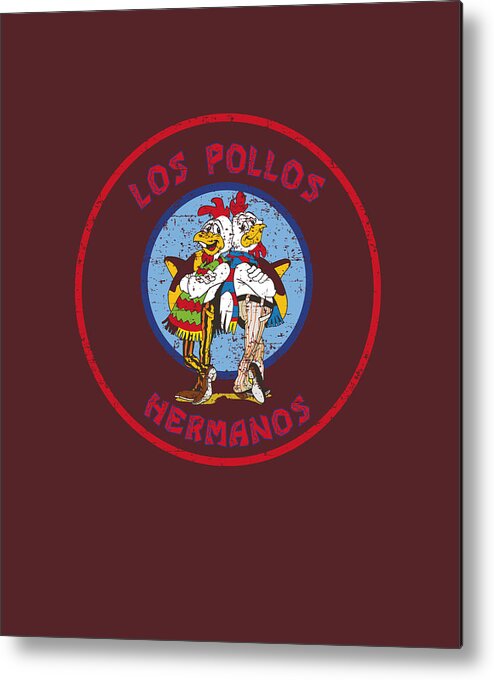The image is a detailed advertisement poster for the Los Pollos Hermanos chicken restaurant. The background is a maroon-red color with an oval shape in the center, also in red. This red oval contains the text "Los Pollos" curved at the top and "Hermanos" curved at the bottom, both in red letters. Inside this red oval is another, smaller, light blue oval with a darker blue outline. Standing in front of this blue oval are two anthropomorphic chickens, dressed in traditional Mexican attire. The chickens, with predominantly white feathers and red accents, stand back-to-back but are looking at each other with smiles. They both have their arms crossed in a confident stance. The chicken on the left is dressed in yellow and black striped pants, a green and red apron, and is holding a large sombrero. The chicken on the right wears a white shirt, gray or beige striped pants, and a similarly large sombrero. Their legs are positioned differently, with one chicken having a leg cocked up and the other having their legs crossed. The detailed illustration captures a festive and traditional aesthetic, emphasizing the cultural theme of the restaurant.